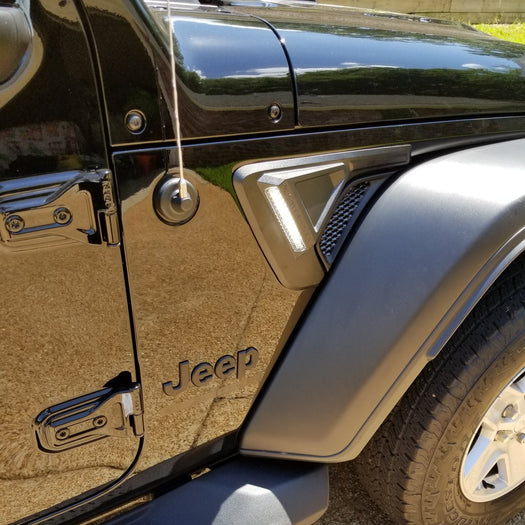This close-up photograph captures a side view of a shiny black Jeep, showcasing intricate details of its front passenger side. The image prominently features a portion of the front right wheel with a silver rim, partially obscured by a gray front tire guard extending over it. The Jeep's hood and fender are visible, along with the iconic "Jeep" emblem displayed on the side of the fender. Large black hinges are noticeable on the door, which also has a raised gray footrail with anti-slip grips, designed for ease of entry. An antenna is visible at the top left of the image, adding to the vehicle’s rugged, functional aesthetic. The vehicle is parked on a gray concrete surface, with a strip of grass faintly visible in front.